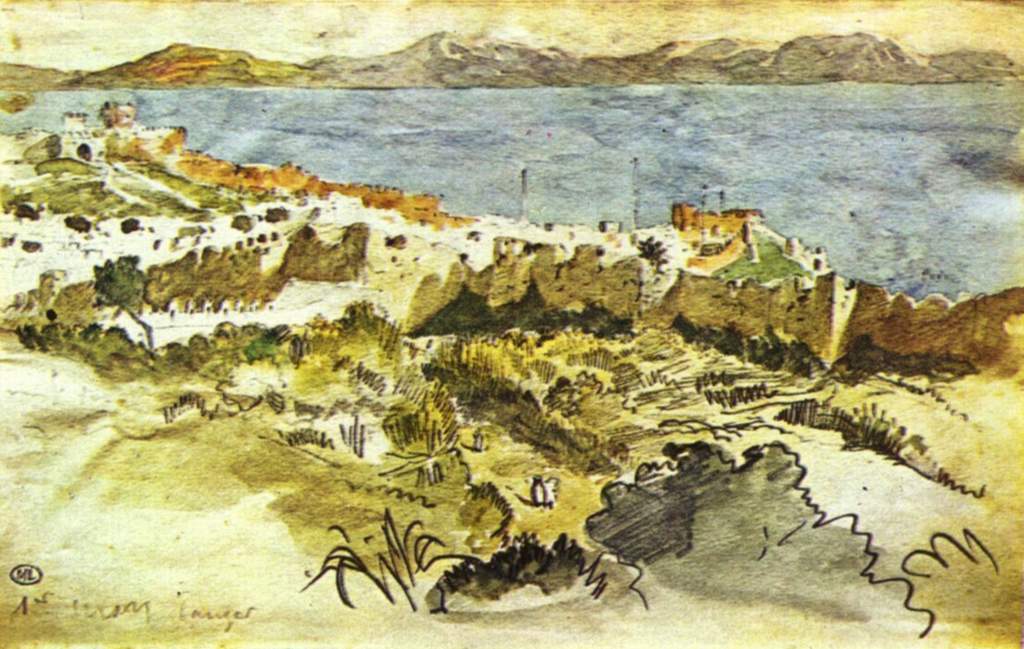In this detailed painting, we are presented with a top-down view of what appears to be an old seaside town, possibly in a desert-like, Californian area. Central to the image is a tranquil body of water, painted in a subtle, faded blue shade that immediately catches the eye. Surrounding this water are tan and brown landscapes dotted with pockets of green grasses and trees, suggesting minimal vegetation due to the arid environment.

The composition includes noticeable structures that resemble castles; one is situated on the upper left side and another in the middle-right section of the painting. These structures are depicted in rust-orange and white hues, adding to the historical feel of the scene. Also apparent is a wall-like formation made of gray stone, enhancing the ancient atmosphere.

The town's buildings vary in appearance but generally display earth tones of brown and beige. Towards the bottom of the painting, a grassy area is visible, with hints of yellow and brown bushes interspersed among some green patches. The background is graced by a row of gray, stony mountains, with one on the left side covered in green, providing a stark contrast to the otherwise desaturated color palette.

The edges of the painting appear faded, almost as if they are burnt, adding to the aged aesthetic of the piece. A partially legible artist's signature can be found on the lower left side, slightly obscured and scratched off, hinting at the artwork's authenticity and antiquity.